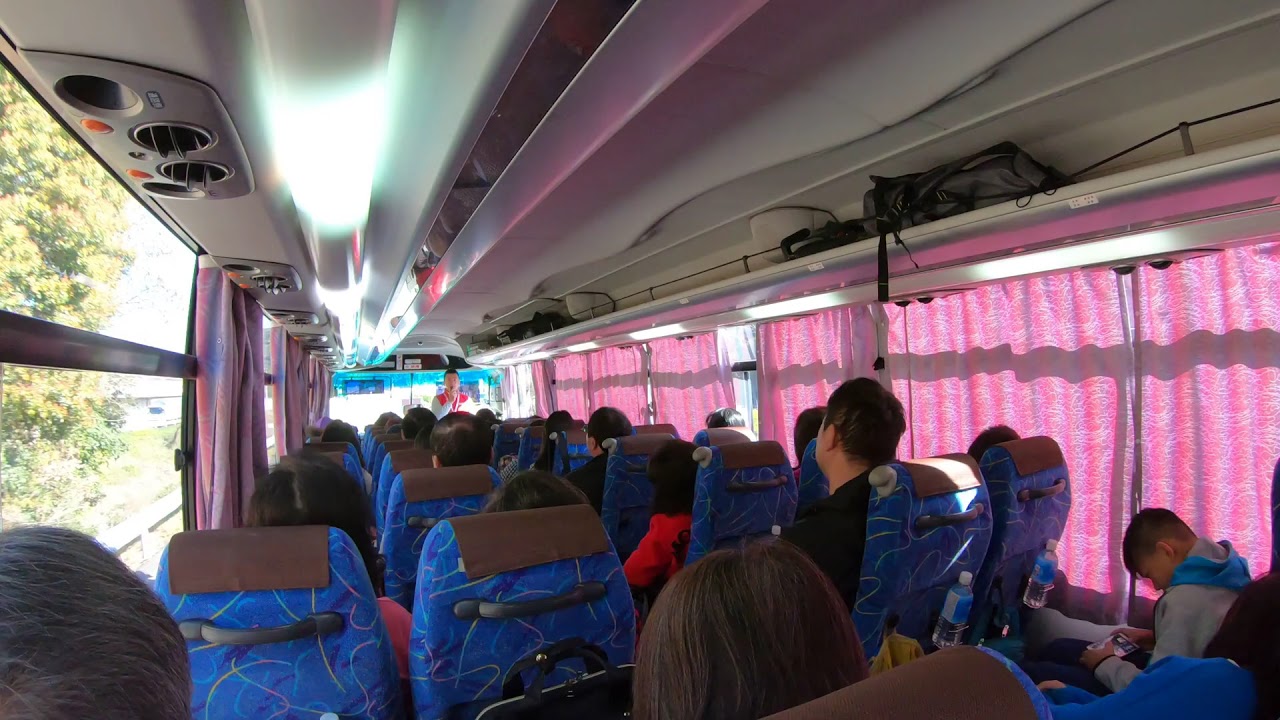The image shows the interior of a large passenger bus, resembling a tour bus often used by groups traveling to destinations like New York City or Washington, D.C. The photo appears to be taken from one of the back seats. The bus seats are predominantly blue with streaks of neon colors and two seats line each side of the aisle. Most chairs have brown fabric tops. At the front, a person dressed in a white and red shirt or vest is speaking into a microphone, presumably giving instructions or providing commentary to the passengers. To the right, some pink drapes cover the windows, with the sun filtering in, while on the left side, the drapes are drawn back, revealing part of a tree and a building outside. The ceiling of the bus is gray with visible ventilation vents. The passengers appear to be of Asian descent, varying in age from children to senior adults. In the bottom right corner, a young boy is engrossed in his phone, possibly playing a game or watching a video.